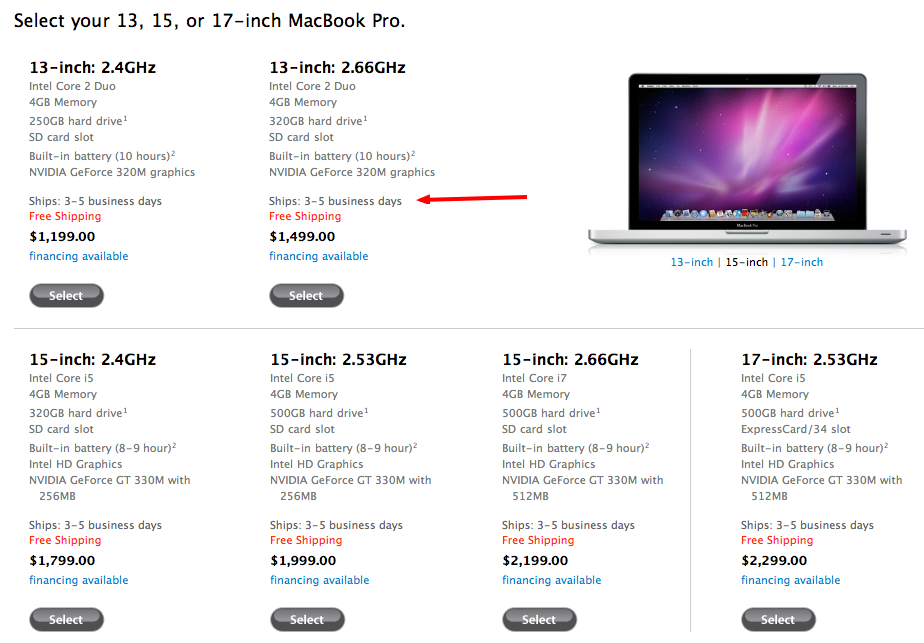This screenshot captures the product selection page for various models of the MacBook Pro. At the top left, there is a section labeled, "Select your 13, 15, or 17 inch MacBook Pro." Below this heading, detailed specifications and prices are listed for each model. 

- **13-inch MacBook Pro models**:
  - The first option features a 2.4 GHz Intel Core 2 Duo processor, 4GB of memory, a 250GB hard drive, and an SD card slot. It is priced at $1199.
  - The second option has a 2.66 GHz processor, and its price is set at $1499. A red arrow is pointing to this model, suggesting that it is the preferred choice.

- **15-inch MacBook Pro models**:
  - The first 15-inch model includes a 2.4 GHz processor and is priced at $1799.
  - The second option offers a 2.53 GHz processor, with a price tag of $1999.
  - The third 15-inch variant features a 2.66 GHz processor and is listed at $2199.

- **17-inch MacBook Pro model**:
  - This model boasts a 2.53 GHz processor, and it is the most expensive option at $2299.

The highlighted 13-inch MacBook Pro with a 2.66 GHz processor seems to be the main focus of interest, likely indicating the user's choice for purchase.